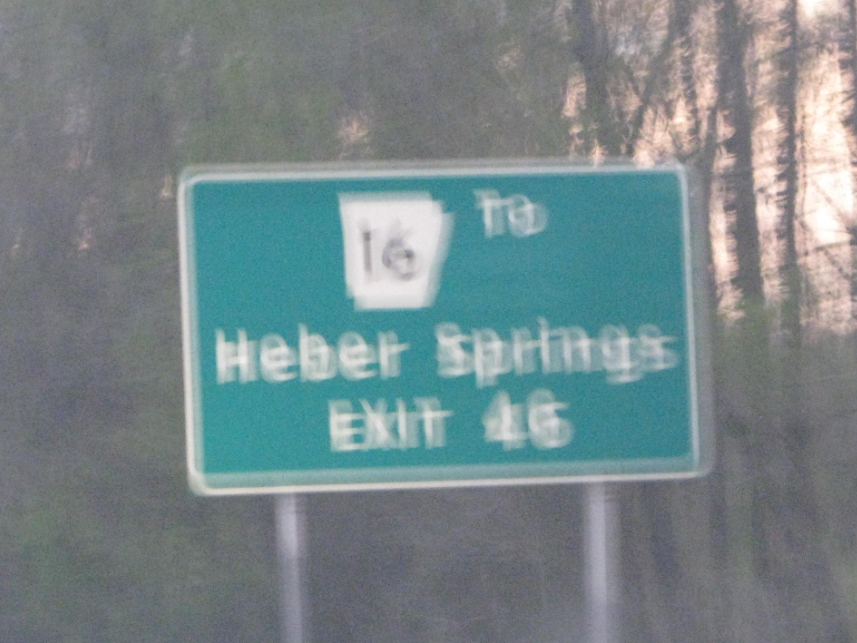This photograph shows a slightly blurry road sign captured on the side of a highway. Dominating the center, the sign features a large green square outlined in white on the inner edge. Towards the upper left corner of this square, there is an emblem that represents the state highway symbol, resembling a square with a slanted right edge. Inside this emblem, in black text, the number "16" appears, although it seems duplicated due to the blurriness of the image. To the right of this emblem, the sign displays a white number "2."

Below the emblem and number, in large, clear white letters, the sign reads "Heber Springs." Further down, it indicates "Exit 46" prominently. The sign is mounted on two gray poles, which are visible emerging from its bottom on both sides. The background consists of a lush forest with green leaves and brown trunks. In the upper right corner, a soft, creamy light filters through the trees, adding a touch of warmth to the scene.